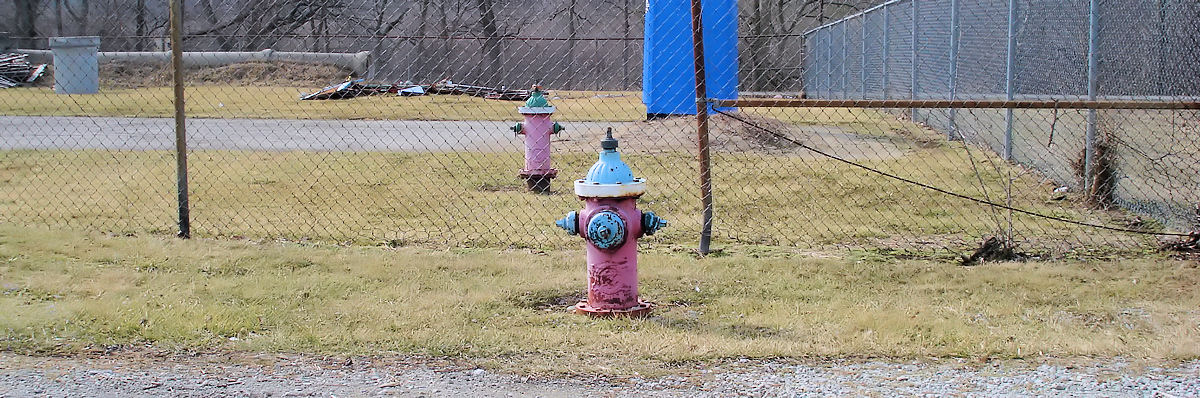This is a wide, panoramic color photograph with a long horizontal frame. The main focus is on a pair of fire hydrants, both located in a grassy area. The grass is predominantly yellow with some patches of green, indicating it needs maintenance. The fire hydrants are primarily red with faded blue or green caps and connectors. Additional detailing includes a yellow band around the top of at least one and a small black screw on top. 

In the foreground, a gravel or blacktop path runs parallel to the grass. Surrounding the area is a chain-link fence, rusty and bent in places, indicating wear and tear. Behind the fence on the right side, there is another fire hydrant similar to the ones in the foreground, and a tall, newer chain-link fence running perpendicularly. 

A blue port-a-potty is visible in the background, partially obscured by the fence. Large sections of cement pipes suggest ongoing construction work. The background also includes a small road or concrete area, with some bare leafless trees visible beyond the fenced perimeter. The detailed description of this scene suggests a place that might be a derelict playground or an unused yard, possibly repurposed for current construction activities.